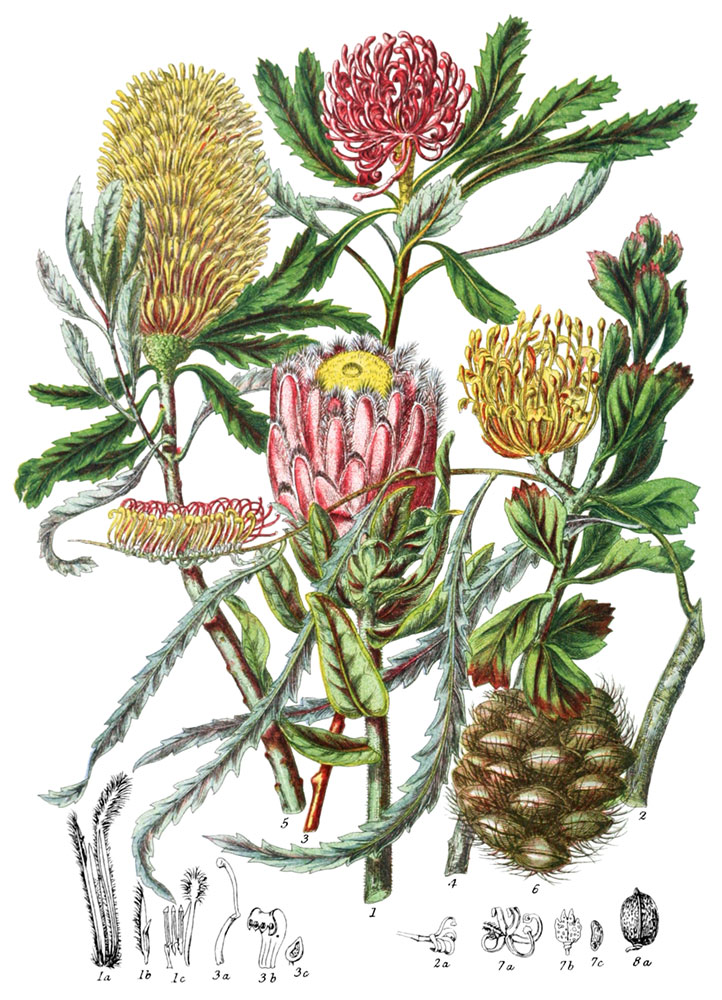This illustration, likely sourced from a botanical field manual or textbook, provides an intricate, hand-drawn depiction of various stages and parts of a plant, possibly a coniferous species. The central focus is a vibrant pink flower with a yellow center, while the top left showcases a striking yellow flower. The lower right corner features a brown pinecone-like seed pod with hair-like structures, resembling clamshells clumped together. Surrounding the flowers are different styles of leaves interwoven among the plant's anatomy, including thin woody stems and cockleburs, suggesting mechanisms for animal dispersal. Below the main illustration are detailed black and white diagrams, labeled with identifiers such as 1A, 1B, 1C, depicting the growth stages of the plant, from seedling to seed production to flowering, characterized by a yellow bushy seed stage resembling a porcupine tail. The entirety of the plant's structure is meticulously labeled with numbers and letters, providing a comprehensive guide to its botanical features.